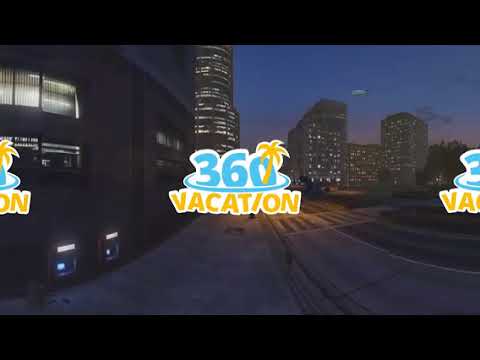The image depicts a nighttime cityscape with a sky transitioning from dark blue to orange, indicating a setting sun. The scene captures an advertising banner for "360 Vacation." The text "360" is stylized in medium blue, with the '0' creatively incorporating a palm tree that extends into the 'I' in "Vacation." The word "Vacation" is presented in bold yellow, all capitalized. This logo appears not only in the center but also partially on the left and right edges of the view. In the foreground, there is a building on the left side featuring two ATM machines at ground level, and white-curtained windows above. Another connected building extends further into the background. To the right, there are multiple tall, illuminated structures with blocky designs. The image also includes a gray sidewalk, a street, scattered trees, and a blimp floating in the evening sky.